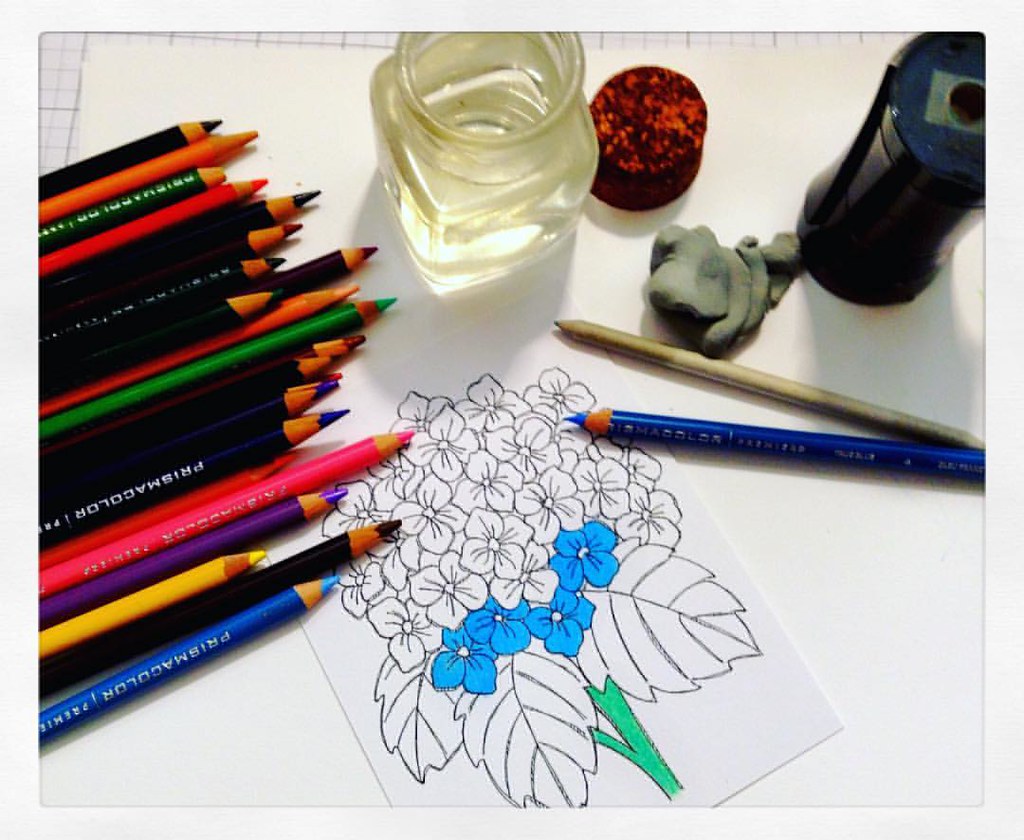This photograph depicts a creatively cluttered art workspace with a partially colored drawing of a flower on a white piece of paper. The drawing illustrates a plant with roughly 15 four-petaled flowers, where the stems and leaves are colored green, and the four bottom flowers are colored light blue. The artwork rests on a piece of graph paper.

To the left of the drawing, there is an assortment of colored pencils, including blue, black, yellow, purple, pink, green, and orange. These pencils are stacked and lined up, indicating a rich variety of colors. On the right side of the image, there are additional colored pencils, approximately 20, laid diagonally and pointing towards the top right corner. Among these, a blue pencil is laid horizontally with a regular pencil positioned above it.

In the upper middle of the picture, there is a jar filled with clear liquid, presumably water, and a red object of indeterminate nature nearby. A thermos is visible at the top right corner, contributing to the scattered yet art-focused atmosphere of the desk. The detailed combination of these elements paints a vivid picture of an active and ongoing art project.